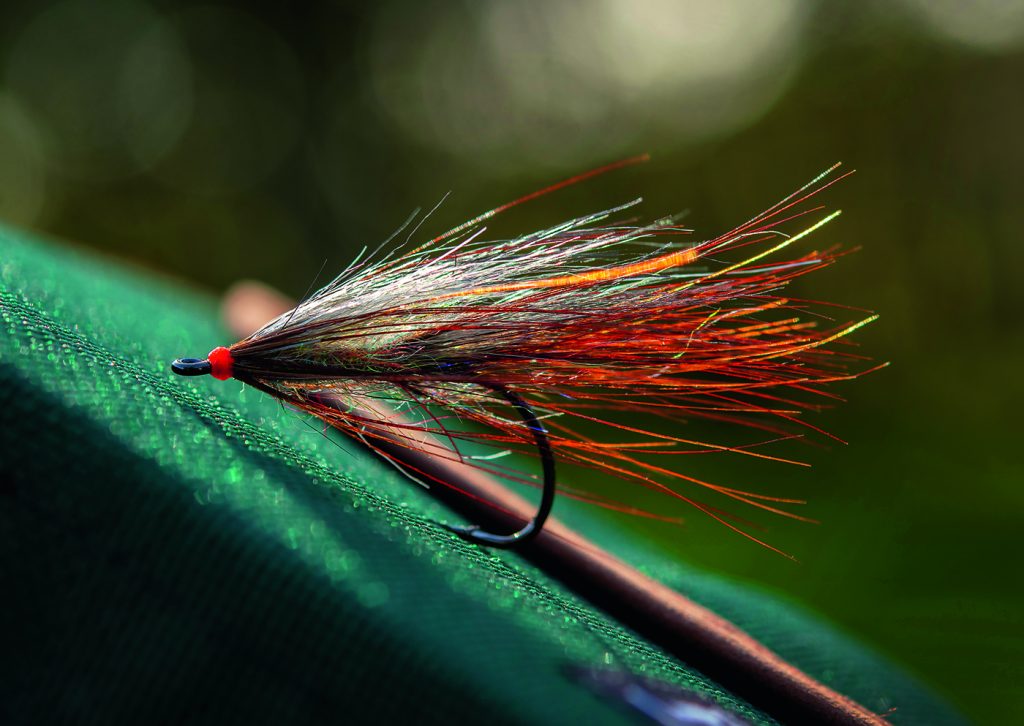The image presents an extreme close-up of the end of a fly fishing rod, showcasing a vividly colored fly fishing lure. The fishing rod itself appears to be thin and dark reddish in color, laying on a green cloth, which might be a forest emerald or darker olive hue. The fly, an intricately crafted object used in fly fishing, features an array of vibrant nylon threads in red, yellow, white, blue, and dark red, along with a small red bead that secures the threads to the hook. The hook, dark navy blue in color, elegantly curves to the right, with its tip pointing backward. The colorful strands of hair extend from the hook, likely designed to attract fish with their flashy appearance. The overall setup, including the partly visible rod, is placed atop the green cloth, enhancing the intricate details and vibrant colors of the fly.